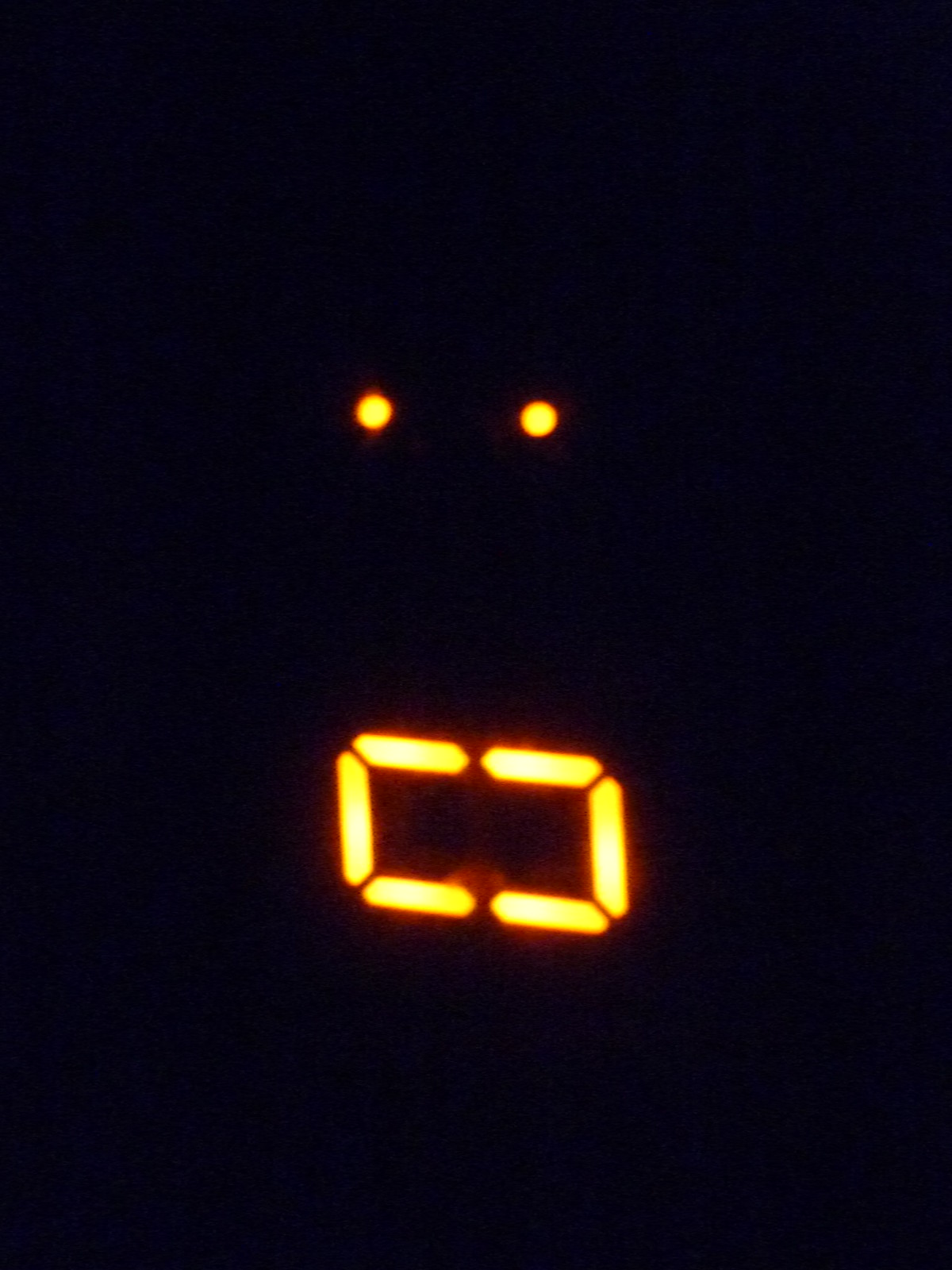The digital image appears to be a sideways orientation of an all-black background featuring a prominent, incomplete numeral '0'. The '0' is distinctly crafted from two vertical lines connected by one horizontal line at the top and one at the bottom. The vertical lines remain unconnected in the middle, leaving a gap where two dots are situated, mimicking the colon often used to separate hours and minutes in time displays. Despite the indication that the device could show time, there are no other numerals present to confirm the actual time, suggesting it could be part of a clock, a scoreboard, or any digital display waiting to convey information.